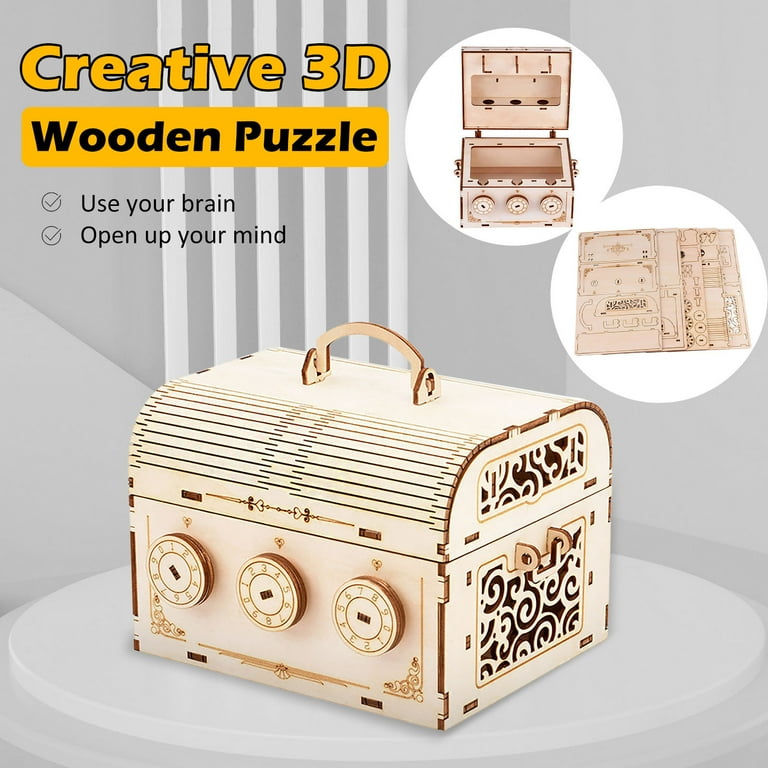This advertisement showcases a 3D puzzle kit that, when assembled, forms an elegant wooden box. The background is grey with subtle vertical white lines. In the top left corner, prominently displayed in yellow lettering, are the words "Creative 3D Wooden Puzzle" followed by the phrases "Use Your Brain" and "Open Your Mind," each with a check mark beside them. The puzzle itself is a light brown, intricately designed box with a handle on top and three numbered dials on the front, resembling a treasure chest or a purse. The sides feature an ornate flower design, adding to its charm. The box sits on a white surface, and its lid can open, revealing its interior. In the top right corner of the image, two circles show detailed images: one of the completed box with its lid open, and the other of the puzzle pieces laid flat, ready for assembly. This visual and descriptive layout emphasizes the sophistication and mental challenge of the puzzle.